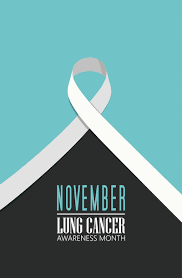The poster, designed for Lung Cancer Awareness Month in November, features a clean, simplistic aesthetic with a rectangular layout. The top half of the image is a soft baby blue, transitioning to a dark black at the bottom. The division between the blue and black sections is strikingly marked by a prominent white ribbon, symbolizing lung cancer awareness, which is lightly shaded to add an artistic touch. The ribbon crosses at the center, providing a visual focal point. Below the ribbon, the words "November" appear in blue text against the black background, followed by "Lung Cancer Awareness Month" in white text, making it clear and distinct. The overall design is minimalist, using flat colors without advanced shading, resembling a postcard in design, effectively highlighting the message without extra detail about the disease itself.